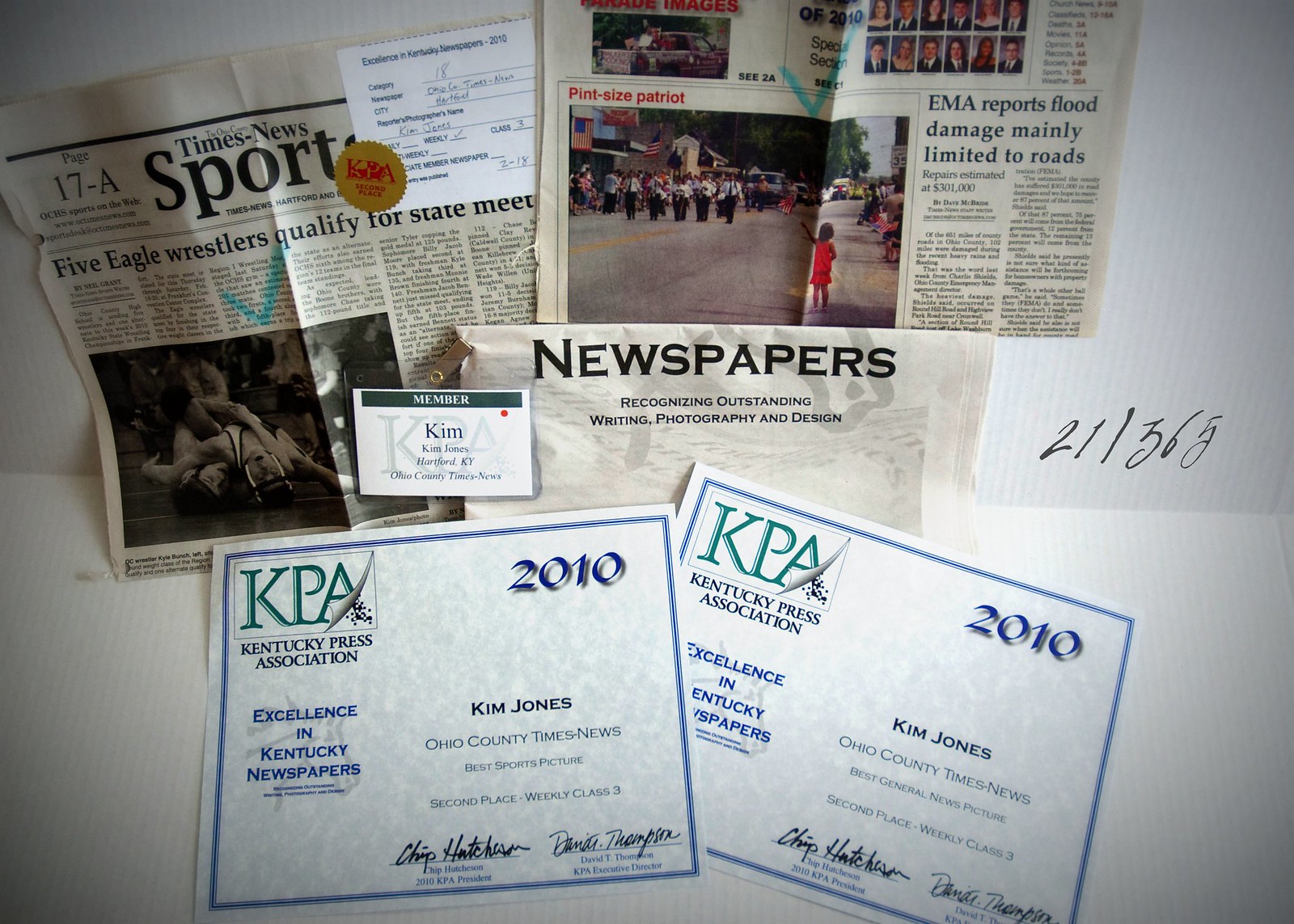This photograph showcases an exhibit displaying a collection of newspaper clippings and awards related to the achievements of Kim Jones in journalism and photography. The focal point includes two prominently featured newspaper pages. On the left, the "Times News Sports" section, dated 17A, highlights an article titled "Five Eagle Wrestlers Qualify for State Meet," accompanied by a faded image of wrestlers. The right page shows people on the street, with the headline "EMA reports flood damage mainly limited to roads," and features a photo captioned "The Tiniest Patriot," depicting a little girl watching a parade.

Below the newspaper clippings, two certificates from the Kentucky Press Association (KPA) are displayed, both awarded in 2010 to Kim Jones of the Ohio County Times News. The certificates recognize Kim Jones for excellence in Kentucky newspapers, specifically for "Best Sports Picture," as evidenced by the photograph of wrestlers. The text and signatures are consistent across both awards.

The arrangement of the items and the positioning on the exhibit wall suggest a curated effort to highlight Kim Jones' contributions and accolades in the field of newspaper journalism and photography. The exhibit label at the bottom, marked "21-365," adds a cataloging element to the display. The overall color scheme includes shades of white, blue, green, gray, black, red, orange, and tan, contributing to the visual narrative of the exhibit.